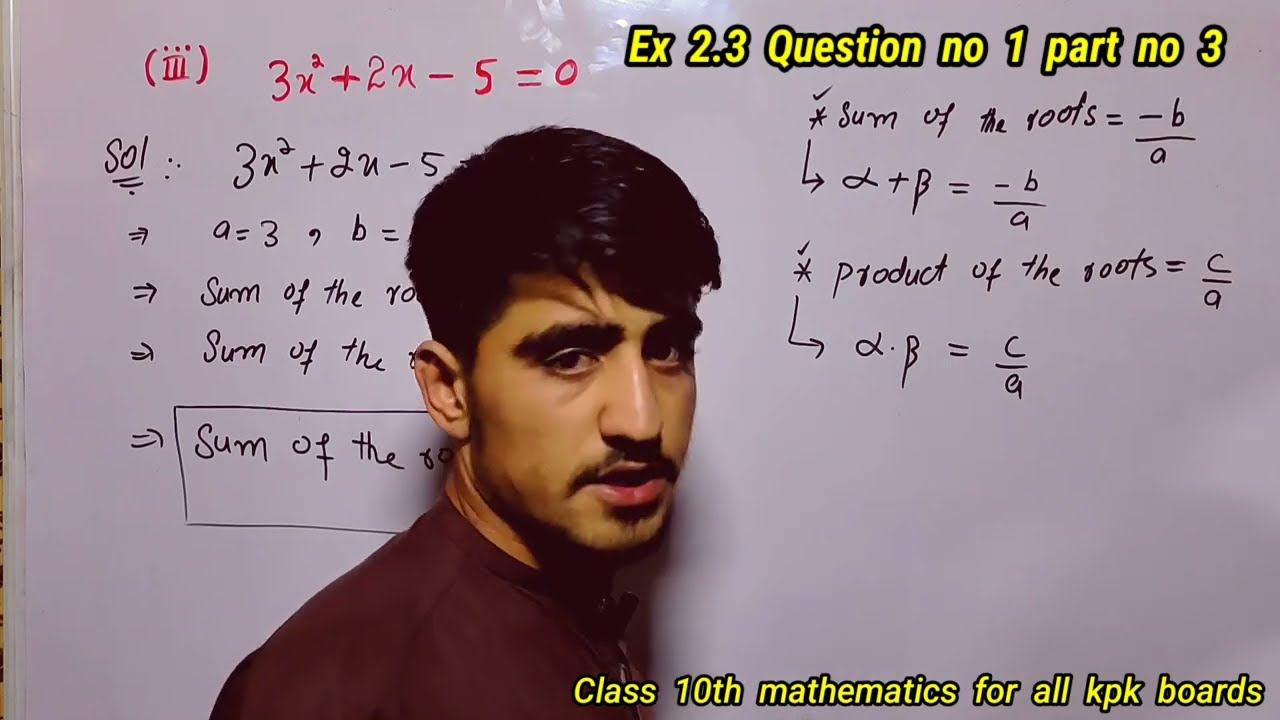In the horizontally aligned rectangular image, a man with short black hair combed to the left, bushy black eyebrows, and a thin black mustache, is standing in front of a whiteboard filled with mathematical equations. He is wearing a maroon T-shirt, and his mouth is open, indicating he is speaking to the camera. The whiteboard is marked with various mathematical formulas written in both red and black. On the left side, a Roman numeral III in brackets precedes a red equation that reads \(3x^2 + 2x - 5 = 0\). Below this equation, partially obscured by the man's head, the word "SOL:" indicates the beginning of a solution. Four steps are listed beneath the equation, but their content is not fully visible.

On the right side of the whiteboard, the title "Example 2.3, Question Number 1, Part Number 3" is clearly visible in yellow letters. Additionally, there is detailed text in the upper right-hand corner, including phrases such as "sum of the roots equals -b/a" and "product of the roots equals c/a," along with various mathematical symbols and arrows. The bottom right corner of the image has the text "Class 10 Mathematics for all KPK Boards" in yellow letters, indicating the educational context of the screenshot, likely from a video of a math lesson. The man, with a serious expression and slightly tilted head, engages directly with the viewer, providing instruction.